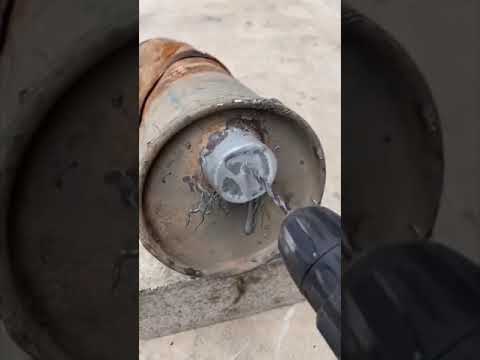This image captures a screenshot from a video, likely posted on TikTok, Instagram, or YouTube, depicting a black drill with a silver drill bit penetrating a rusty, metal cylinder. The worn and corroded cylinder, which appears to be partially recessed and spotted with white residue, is positioned on a grey concrete surface. The backdrop of the image is indistinct, potentially featuring ground or dirt. The scene suggests a vintage or worn-out industrial setting. The drill is seen boring into the cylindrical object, which evokes the look of a smaller, oxidized oil drum laid on its side. This central action fills the frame, drawing attention to the interaction between the drill and the deteriorated metal. The image might be part of a social media post, as suggested by the layout and appearance.